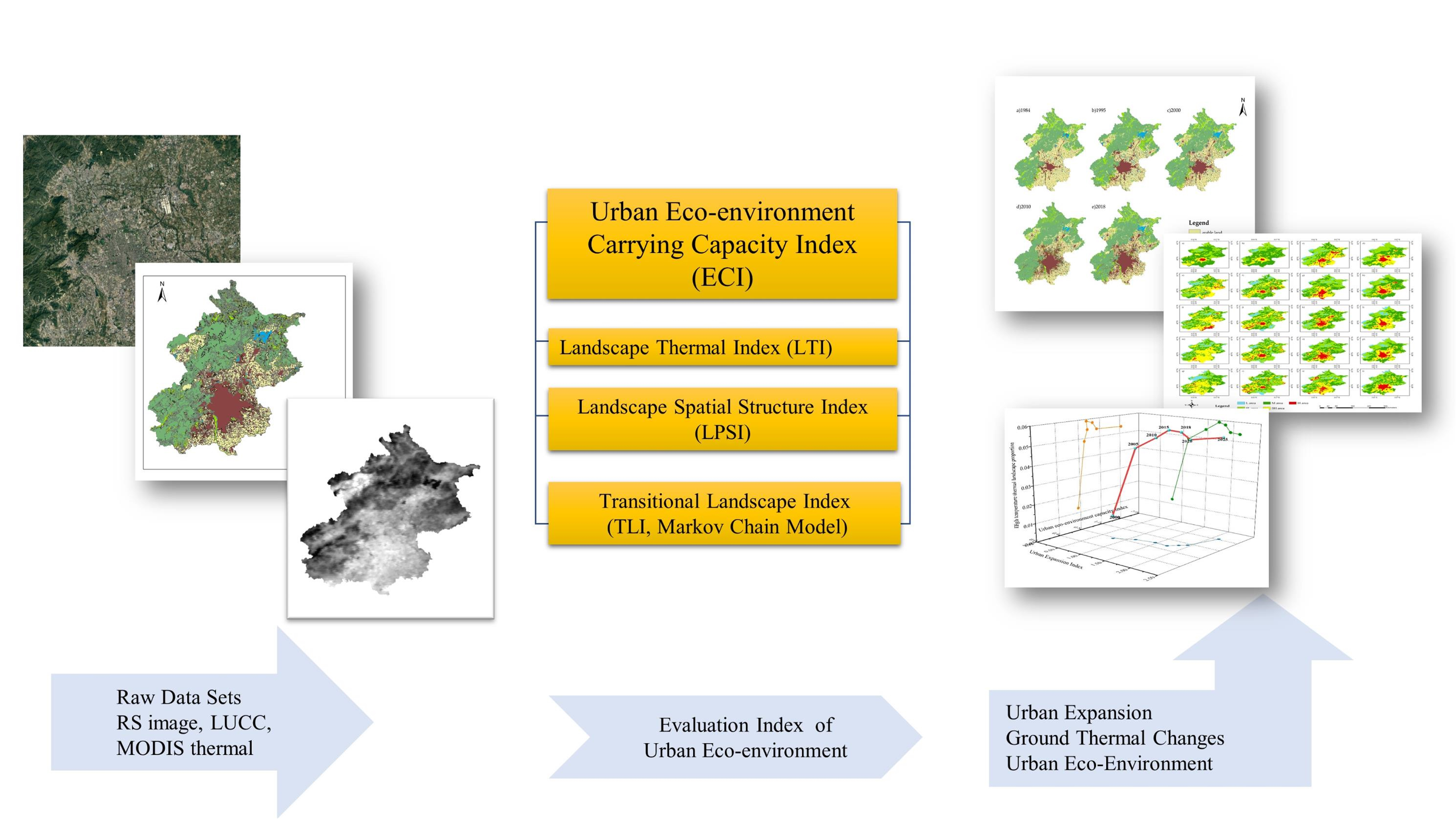This horizontal image, which extends beyond any defined exterior boundary, is a detailed flow chart featuring various illustrations and textual information. It lacks a title but provides a comprehensive breakdown of urban eco-environment analysis processes. At the left bottom corner, a gray arrow with black text indicates "Raw Data Sets, RS Image, LUCC, MODIS Thermal." Directly above this, there are three diagrams or computer-generated prints.

Moving to the center of the flow chart, a second gray arrow labeled "Evaluation Index of Urban Eco-Environment" points upward towards four yellow rectangles. Each rectangle contains black text, listing significant indexes: "Urban Eco-Environment Carrying Capacity Index (ECI)," "Landscape Thermal Index (LTI)," "Landscape Spatial Structure Index (LPSI)," and "Transitional Landscape Index (TLI) Markov Chain Model."

On the right side, a third gray arrow labeled "Urban Expansion Ground Thermal Changes, Urban Eco-Environment" suggests the resulting impacts and changes on the urban eco-environment. Above this arrow, additional diagrams enhance the visual representation of the processes described in the flow chart. Collectively, the image intricately details the structured evaluation of urban eco-environmental factors and their thermal dynamics.